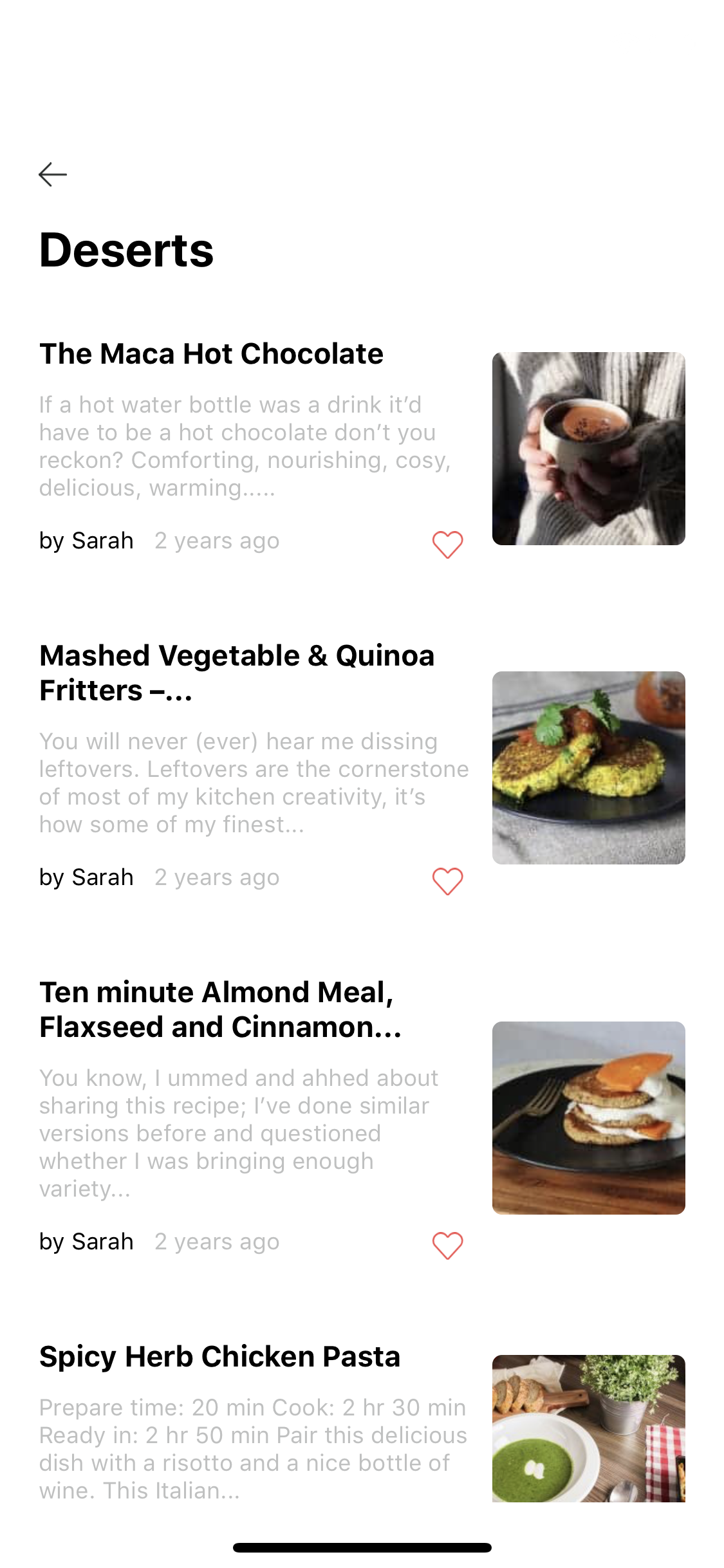The image displays a long, vertically-oriented page, likely captured from a phone screen. The text is predominantly in black, with a larger font at the top announcing "Desserts." Below this header, in black letters, is the title "Maca Hot Chocolate," accompanied by a brief description in gray text beneath it. To the right of this text, there is an image of hands holding a cup of hot chocolate. 

Following this, there are three additional sections, each featuring a different dessert. The first section highlights "Mashed Vegetables," with an accompanying image depicting mashed vegetable fritters. The next section is titled "10-Minute Almond Meal Flaxseed and Cinnamon," and to its right is an illustrative photo of the dish. The final section features "Spicy Herb Chicken Pasta," with an image of the pasta dish situated to the right.

Each dessert title is followed by a description underneath, and all entries conclude with a note that they were posted by Sarah two years ago.